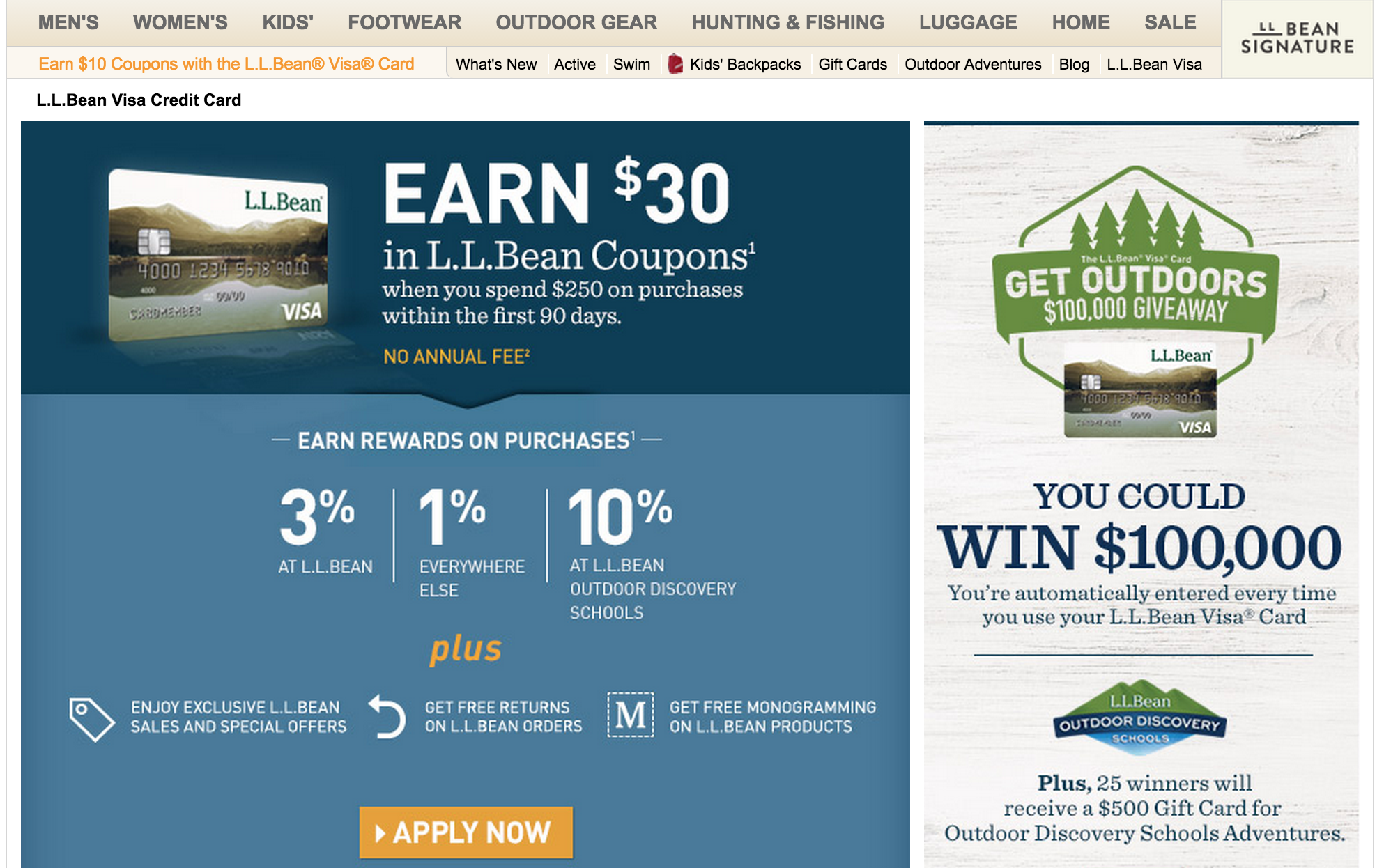The web page prominently features a navigation bar at the top, categorized into men's, women's, kids', footwear, outdoor gear, hunting and fishing, luggage, home, and sale sections. On the right side of the header, it displays 'L.L. Bean Signature,' indicating the website's name. 

Directly below the navigation bar, there is an announcement promoting a $10 coupon offer with the acquisition of an L.L. Bean Visa card. Adjacent to this, users can explore various options such as 'What's New,' 'Active,' 'Swim,' 'Kids Backpacks,' 'Gift Cards,' 'Outdoor Adventures,' 'Blog,' and details about the 'L.L. Bean Visa.'

The main content is divided into two significant sections. The larger left section advertises an enticing offer: earn $30 in L.L. Bean coupons when spending $250 within the first 90 days using the L.L. Bean Visa card. The image alongside the text features the Visa card, emphasizing additional benefits like no annual fee, 3% rewards on L.L. Bean purchases, 1% on all other purchases, and 10% rewards at L.L. Bean Outdoor Discovery Schools. Cardholders also enjoy exclusive sales, special offers, free returns on L.L. Bean orders, and complimentary monogramming on their products. An 'Apply Now' button is provided for immediate action.

On the right, there's a promotion for the 'Get Outdoors $100,000 Giveaway,' which highlights a significant prize structure. By using the L.L. Bean Visa card, users are automatically entered for a chance to win $100,000. Additionally, 25 winners will be awarded a $500 gift card for Outdoor Discovery Schools adventures. This section is adorned with an image of the gift card for visual emphasis.